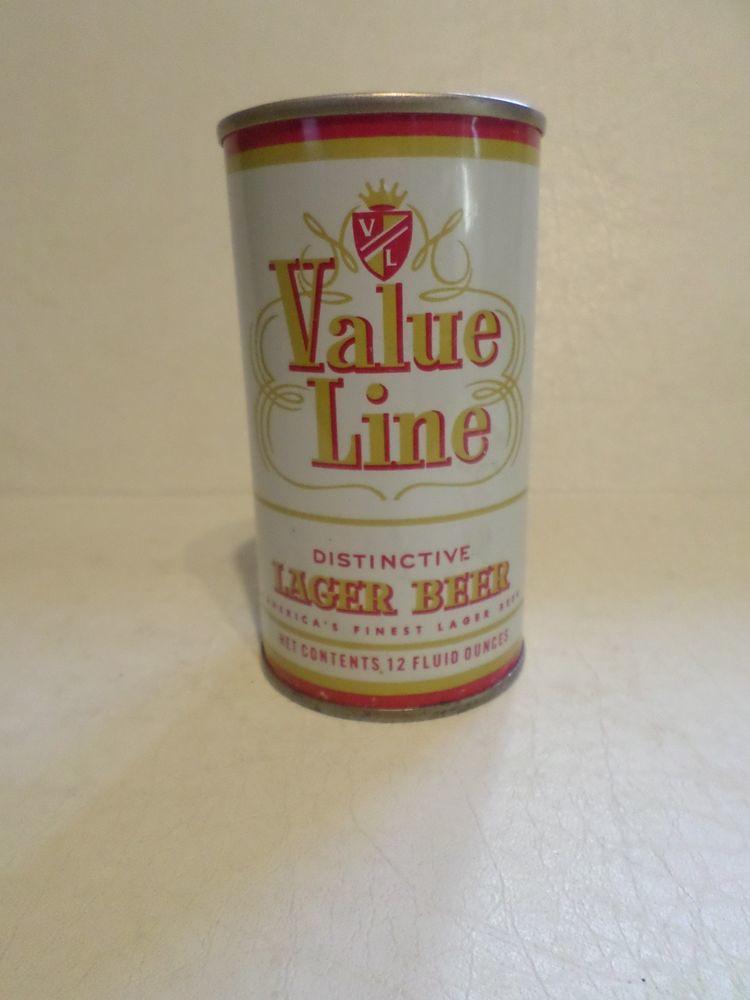This image features a carefully staged photograph of a vintage beer can against a pristine white backdrop. The can itself is predominantly white, adorned with intricately designed gold and red lettering. At the top, a distinguished shield bearing the initials "VL" and crowned with a regal emblem captures immediate attention. Below this emblem, the name "Value Line" is prominently displayed in gold and red hues. Further down, the text "Distinctive Lager Beer" denotes the type of beverage. While some additional text beneath this is illegible, the can clearly states "Net Contents 12 Fluid Ounces" near the bottom. Completing the can’s design, there are horizontal bands of gold and red, adding a touch of elegance to its vintage appeal.